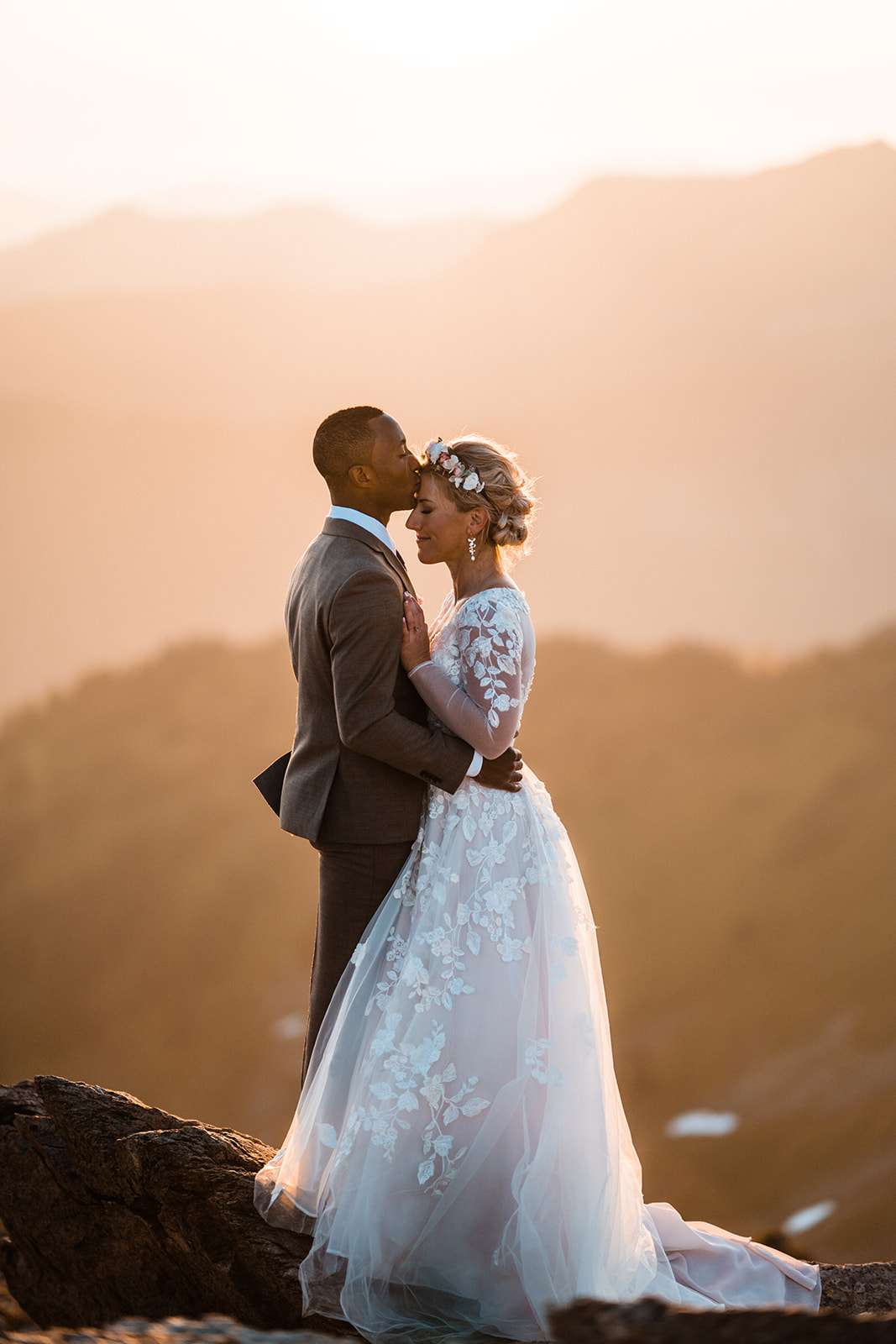This professional, vertical wedding photo captures a heartfelt moment between the bride and groom as they stand on a giant boulder overlooking a blurred, mountainous valley at sundown, casting an orange tint over the scene. The African-American groom, with closely cropped hair, is on the left, dressed in a light brown or taupe suit paired with a white shirt. He tenderly places his right hand on the waist of his blonde, Caucasian bride, who is on the right. She wears a flowing white wedding dress adorned with lace and floral print, her eyes gently closed with a slight smile as he kisses her forehead. Her left hand rests on his chest, and she has flowers in her hair, adding a delicate touch to her look. Both are turned slightly in profile, sharing a chaste embrace that captures the intimacy and joy of their special day.